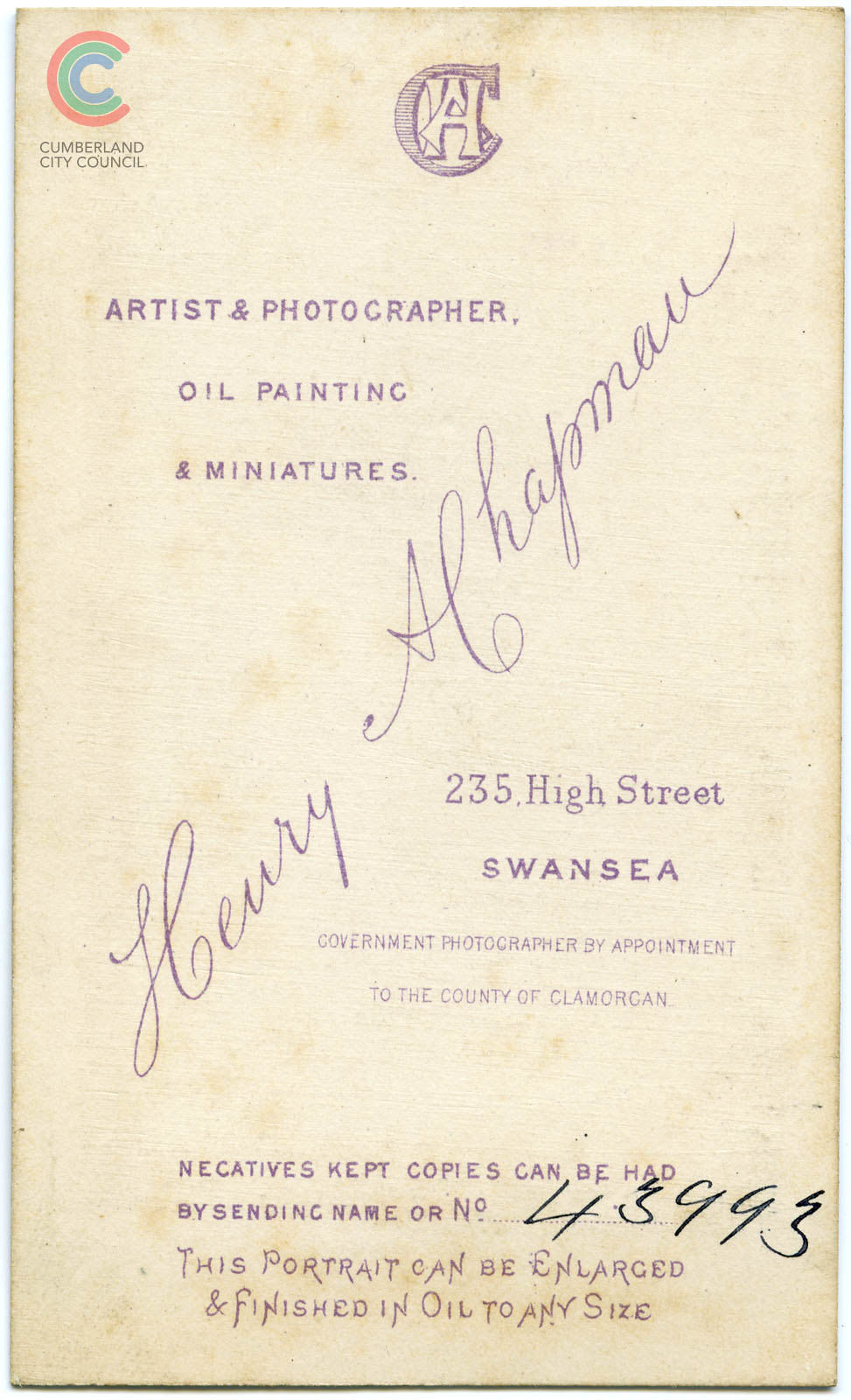This image is a vintage, rectangular book or magazine cover, approximately six inches tall and three inches wide, with a cream-colored background marked by some yellow staining. In the upper left-hand corner, there is a distinctive logo for the Cumberland City Council, consisting of three concentric letter C's in blue, green, and red. Beneath the logo, "Cumberland City Council" is printed in black. In the central upper portion, there are large, intertwined letters "C," "H," and "A," with the "C" encircling the other two.

The main text on the cover is printed in light purple and reads, "Artist and Photographer, Oil Painting and Miniatures." Diagonally across the cover, in cursive handwriting, it says "Henry A. Chapman," though the surname is somewhat hard to read. Below this, in printed text, it states, "235 High Street, Swansea, Government Photographer by Appointment to the County of Glamoragn." Further down, it notes, "Negatives kept, copies can be had by sending name or number," with the handwritten number "43993" in black ink. At the very bottom, it concludes with, "This portrait can be enlarged and finished in oil to any size."